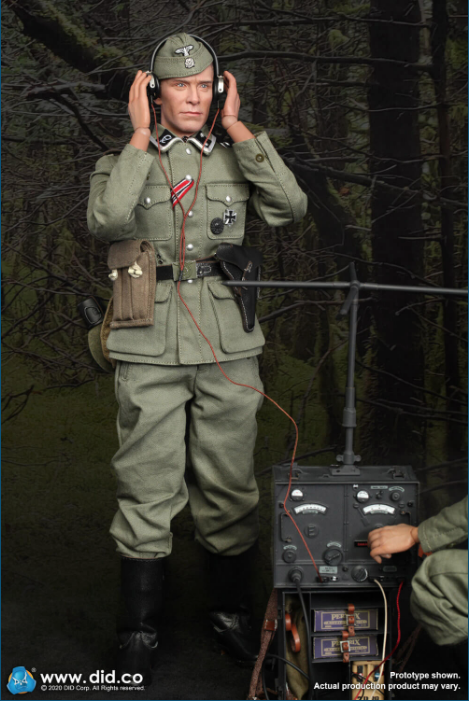The image from www.did.co features a highly detailed action figure of a World War I-era German military officer. The figure is dressed in a green uniform complete with black boots, a tactical waistband, and a distinct hat. A black German cross is prominently displayed on the left shirt pocket, signifying his rank and allegiance. The soldier is holding onto a pair of headphones, which are connected by a long red wire to a large grey radio unit on the ground. Adjacent to this soldier, on the right side of the image, another figure's hand and part of his leg are visible; this figure appears to be adjusting the knobs on the radio device, possibly altering its frequency. An antenna rises from the radio, affirming its role as a communication device. In the background, trees add a touch of environmental realism, framing the military scene. The bottom of the image includes the notice, "Prototype shown. Actual production product may vary," indicating that this might be a catalog photo or a part of an instruction manual.